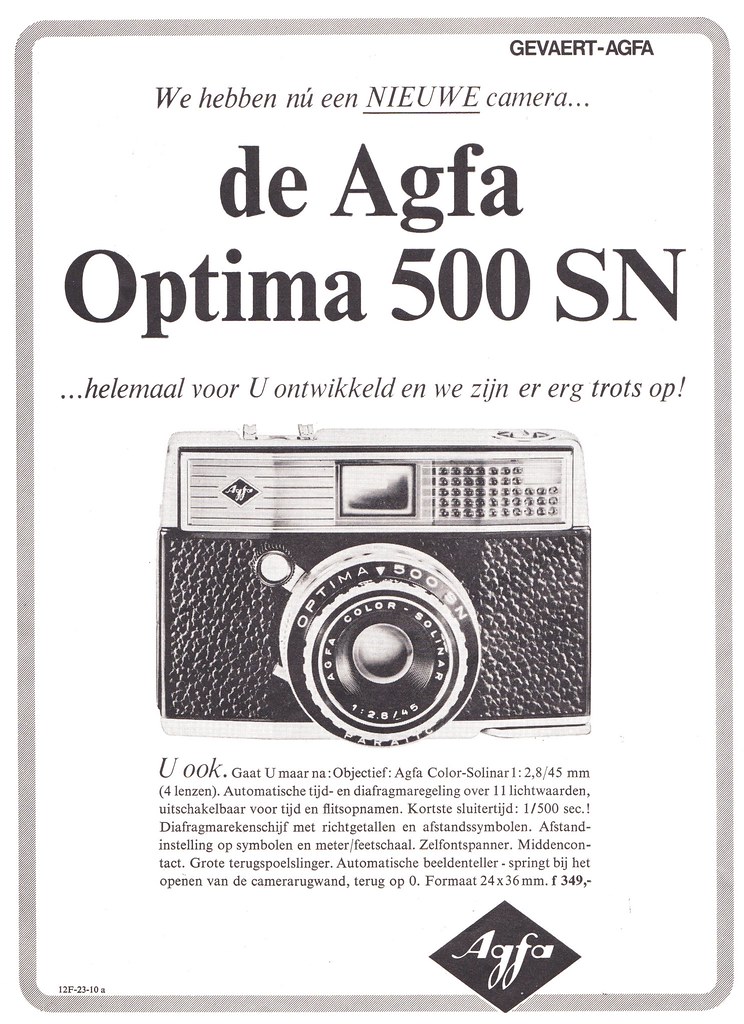The image depicts a vintage advertisement for a rectangular, black and silver camera set against a bright, clear backdrop. The black and white ad prominently features the camera model "Optima 500SN" and the brand name "Agfa Color Solenar" above its lens. The camera's front boasts a black textured area akin to leather, while the top part displays horizontal grooves on the left and several small circles on the right, likely the flash, accompanied by a black diamond-shaped logo with "Agfa" in white letters.

At the top-right corner of the ad, the words "Gewert-Agfa" are displayed in dark gray. Below this is a slogan written in a different language, likely German or Dutch, stating "WE HEBBEN NU EEN NIEUWE CAMERA." Further down, in larger gray text, it reads "De Agfa Optima 500SN." A concise paragraph of specifications follows underneath the camera image, concluding with the Agfa diamond logo positioned at the bottom-right corner. The overall layout is clear and bright, making the details of this classic advertisement easily discernible.